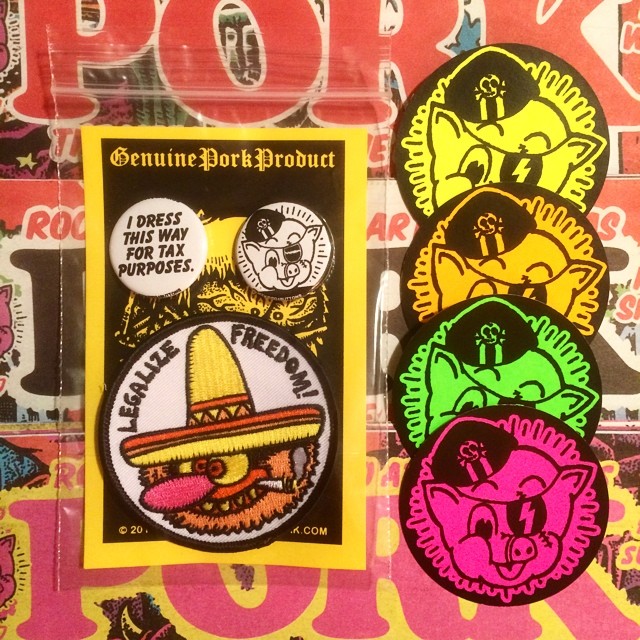This photograph showcases a collection of sew-on patches displayed against a shop window with the word "PORK" in bold red letters at the top. On the left side, three patches are enclosed in a clear plastic Ziploc bag: the first is a round patch with black text stating "I dress this way for tax purposes," the second is another round patch depicting a cartoon pig with an eyepatch, and the third is a larger circular patch featuring what appears to be a monster-like character resembling Gonzo from the Muppets, adorned with a Mexican sombrero and a cigarette-like object in its mouth, accompanied by the phrase "Legalize Freedom." To the right of the bag are four more round patches stacked partially on top of each other, each displaying the same cartoon pig with the eyepatch, skull-adorned biker hat, and a scar, but in different vibrant colors: bright pink, bright green, bright orange, and bright yellow. The background details include the visible words "Genuine Pork Product" and "Pork" in various places, contributing to the quirky and eclectic theme of the display.